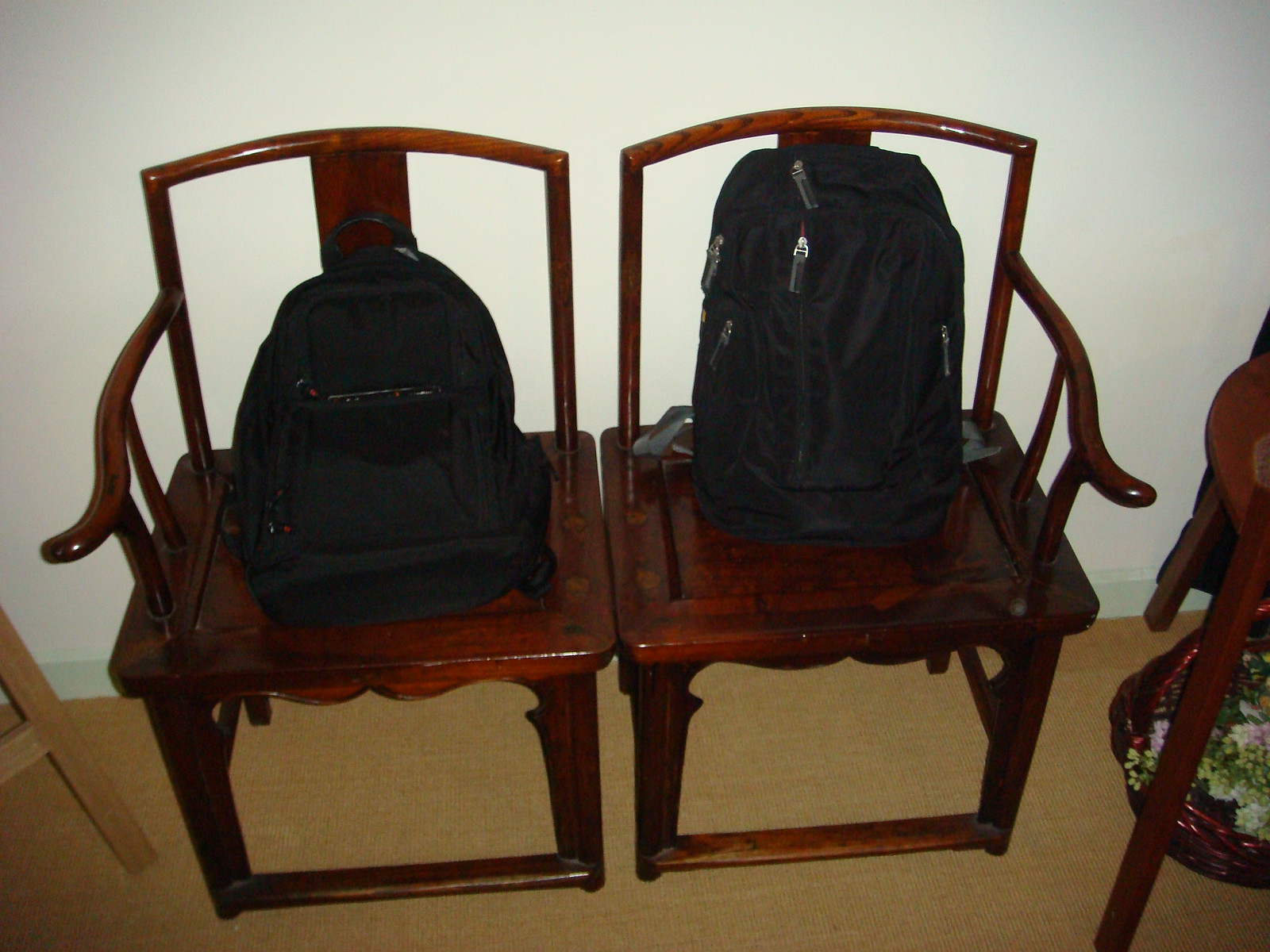This image features two dark cherry brown wooden chairs, each supporting a black backpack, possibly of the kind used by schoolchildren. The chairs, distinguished by their single armrests and open back framed with a wide central slat, are placed adjacent to one another. They are situated in a room with a beige wall and a flat brown carpet. On the left side of the chairs, part of an easel's A-frame leg is visible, contributing to the cozy, arranged setting. To the right, the edge of a wooden coffee table can be seen. Additionally, a wicker basket with floral decorations rests nearby, enhancing the cozy ambiance of the room.